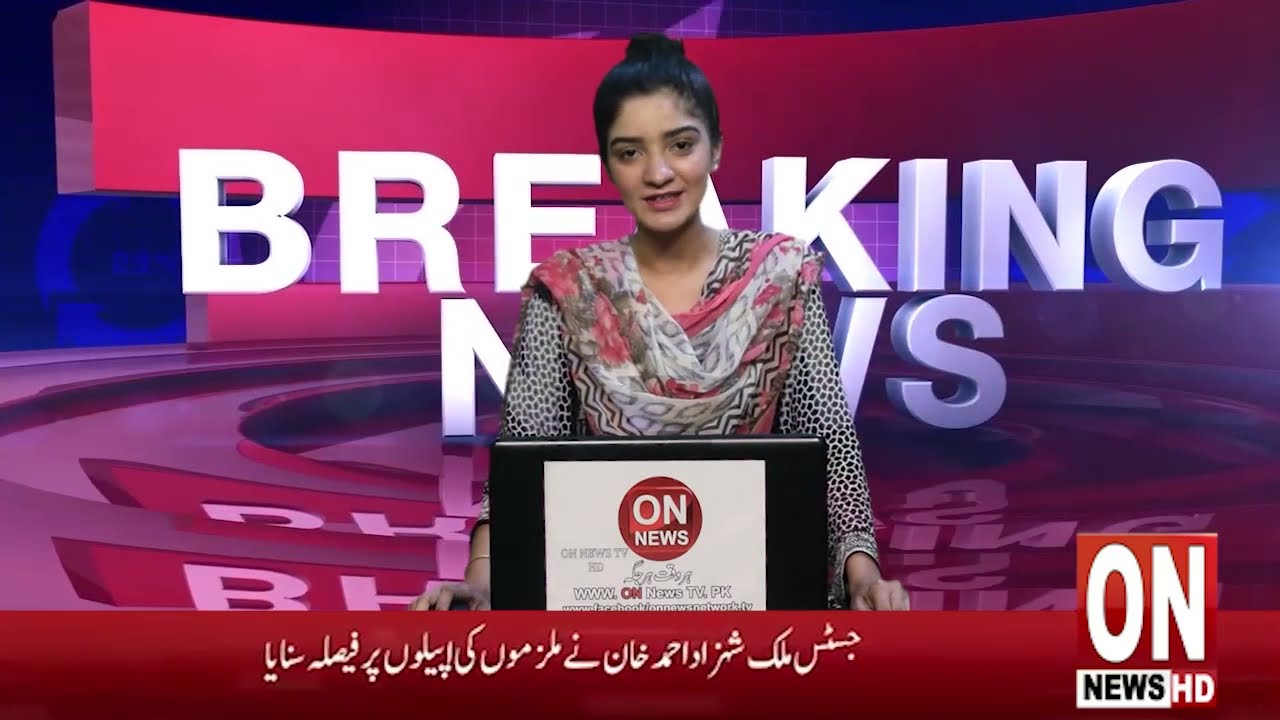The image is a horizontal rectangular frame showcasing a woman on a news show. The woman, who appears to have slightly darker skin and dark hair pulled up into a bun, stands centrally. She's adorned in a blouse with cheetah print sleeves and a black and white pattern, accented by a red, gray, and white patterned scarf or shawl around her chest and neck area. She is positioned in front of a digital screen displaying the words "BREAKING NEWS" in large white block letters, partially obscured by her body. The background integrates a circular pattern with red, blue, and purple hues. At the bottom of the image, a horizontal red strip features white symbols, and in the lower right corner, it reads "ON NEWS HD," with "ON" in white capital letters and "NEWS" in black capital letters. On the center-left of the image, another screen or possibly a laptop displays a logo or text reading "ON NEWS" inside a red circle. The scene conveys a live broadcast setting, likely from a news studio.